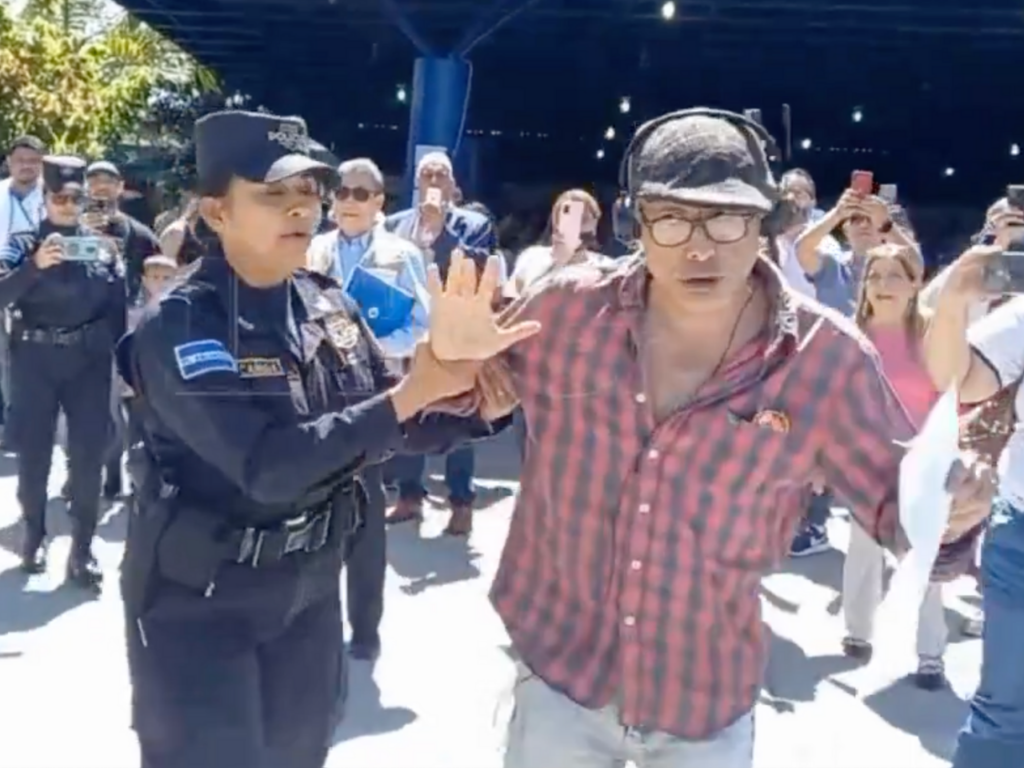In the photograph, a woman in a blue police uniform with a black belt and several patches, including one on her right shoulder and various others on her chest, stands prominently in the foreground on the left. She wears a square-shaped blue cap featuring white writing on the front, and extends her arms to the right, holding the forearm and back of a man standing beside her. The man, dressed in a red and black plaid button-down shirt, blue jeans, a gray cap, and headphones over his ears, has light brown skin, brown glasses, and holds a long piece of paper in his left hand while something protrudes from his left shirt pocket. His right hand is open and extended forward. Behind this pair, a crowd of onlookers, including another person in uniform, stands, many capturing the scene with their cell phones. The background reveals an outdoor setting bathed in sunlight, with a grayish-white hardtop surface underfoot, the overhang of a stadium visible to the right, and a faint glimpse of a tree and enclosure with lights in the distance.